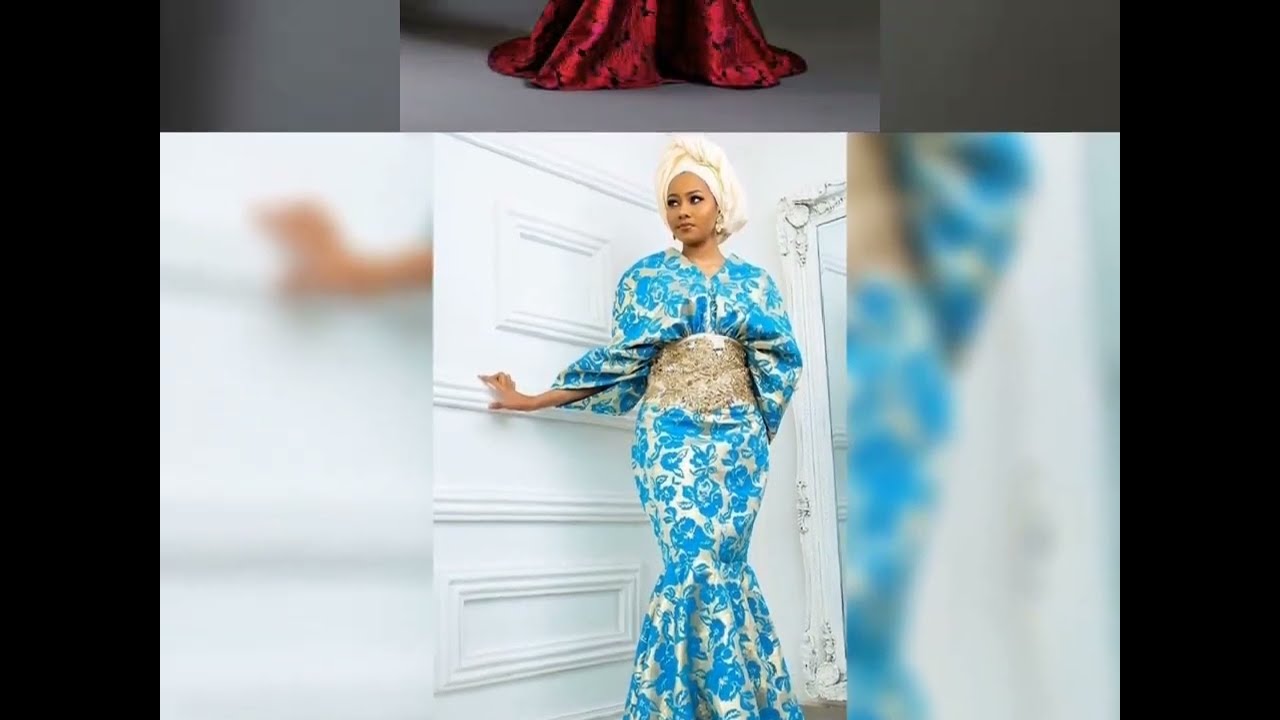The image features a young, dark-skinned woman modeled in a striking white and turquoise blue floral kimono-style dress. Her dress, made of a high-quality, slightly shiny material, features an ornate blue floral pattern and a prominent light brown belt around her midsection. She is adorned with heavy makeup and elegant dangling earrings. Her head is wrapped in a white fabric, somewhat akin to a turban, and she stands against a white wall with wooden features. The scene is partially blurred, with clearer focus on the woman at the center, who extends her right arm for support while gazing off to her right. The background also includes an ornate white-framed mirror, enhancing the sophisticated setting, suggesting this could be part of a fashion video. The top of the image also shows a transition effect, revealing the bottom of a red dress at the very top.